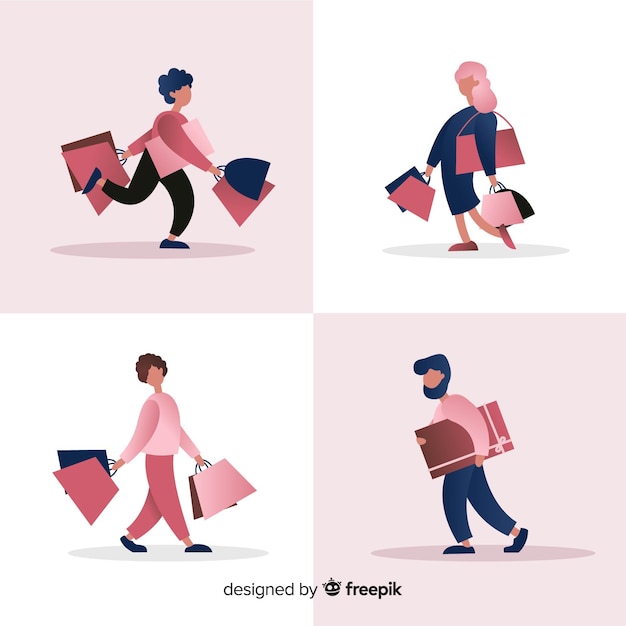This square image, divided into four quadrants, is a simple yet vibrant illustration by Freepik that captures the theme of people shopping. Each quadrant showcases a different figure in bold, basic colors with minimal details, emphasizing the dynamic activity of shopping.

In the top left quadrant, set against a blue background, a woman with curly blue hair and a pink shirt is running, carrying shopping bags in both hands and a box tucked under her arm. The top right quadrant, with a white background, features another woman in a black or blue dress, with a pink purse over her arm and pink hair, also holding shopping bags in both hands. 

The bottom left quadrant, also with a white background, depicts a figure with short brown hair, dressed in a pink long-sleeve shirt and pants, walking while holding shopping bags. Finally, the bottom right quadrant, against a pink background, shows a man with blue hair and a blue beard, wearing a pink shirt and blue pants, walking to the left with a large pink gift under his arm. 

Throughout the illustration, all the characters are engaged in various stages of shopping, creating a lively and cohesive scene.